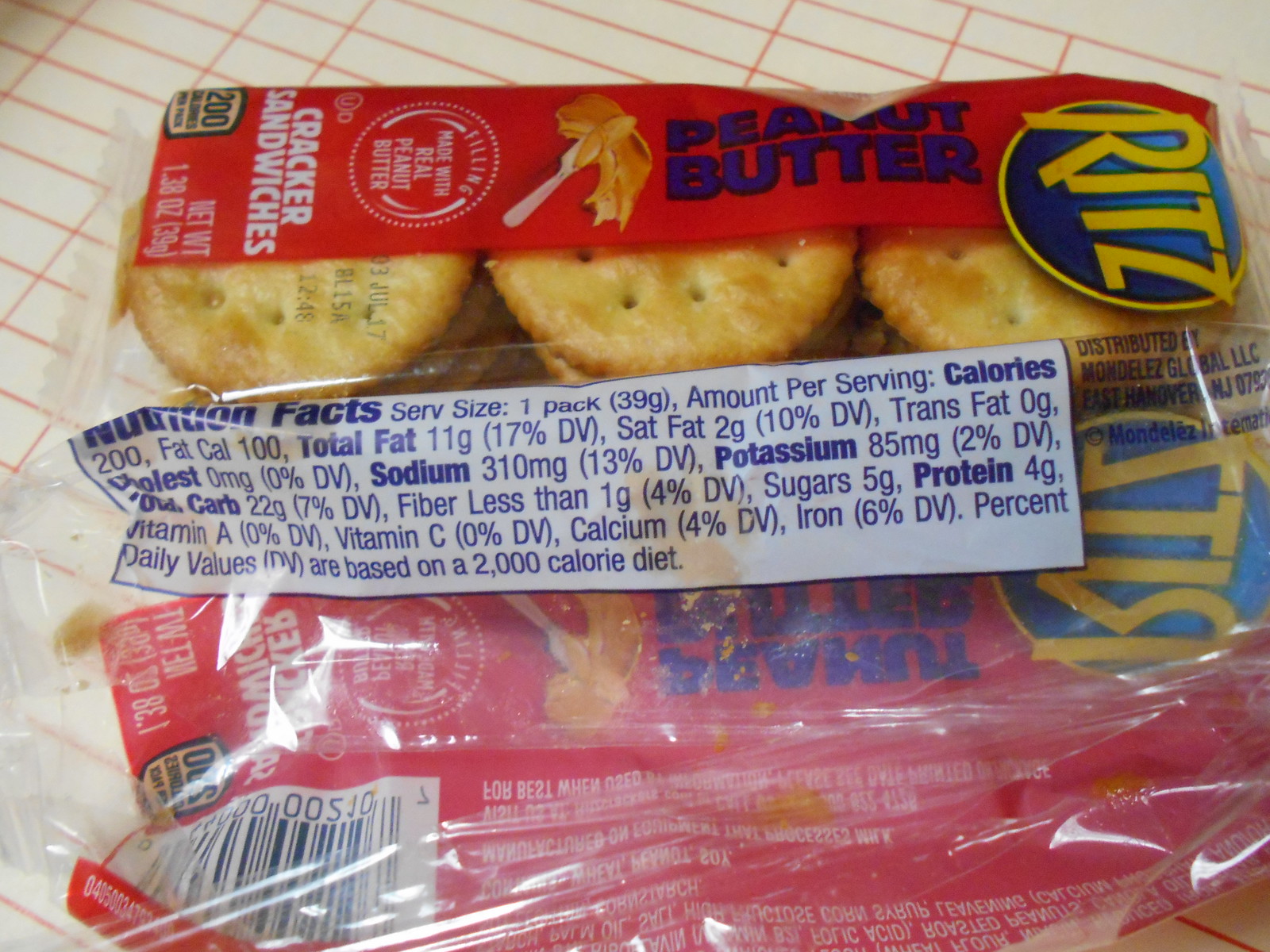This close-up, horizontally oriented photograph depicts a small, clear package of Ritz peanut butter cracker sandwiches resting on a white table adorned with orange lines resembling those in a notebook. The package features a prominent red section with the words "peanut butter" in blue lettering. Above this, a dark blue circle displays "Ritz" in yellow letters. Adjacent to the word "peanut butter" is an image of a plastic knife smeared with peanut butter. Lower on the package, a white label on the red background reads "cracker sandwiches" in white letters. The nutrition facts are prominently displayed in the center of the package, detailing serving sizes, calories per serving, and various nutritional information such as fats, cholesterol, sodium, potassium, vitamins, and protein. The package contains six peanut butter cracker sandwiches and displays a UPC code at the bottom, visible through the clear plastic. An unopened package lies next to an empty, opened one on the table.